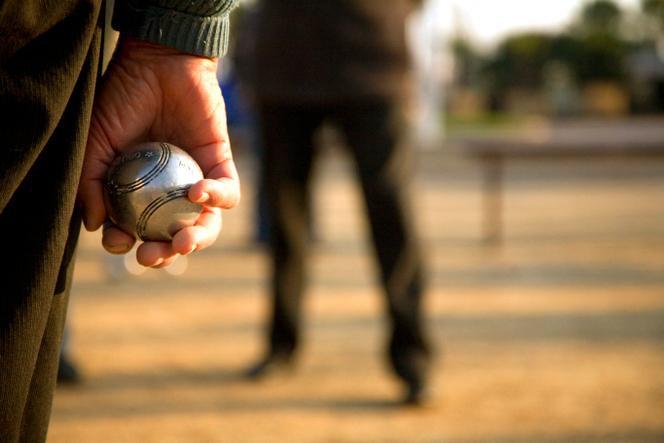In this mostly out-of-focus photograph, the clear portion on the very left-hand side shows a man's hand, palm facing the viewer, wearing a green sweater with the sleeve visible down to the wrist, where the image cuts off. His hand is clutching a bright silver object resembling a baseball, made of metal with visible seams. He appears to be wearing dark-colored, possibly green, pants. In the center of the image, another man can be seen from the waist down, clad in what seems to be brown or dark pants, with his figure remaining blurry and out of focus. The indistinct background likely depicts a sports ground, possibly a baseball field, with a man in what might be armor or a detailed outfit standing ambiguously in the distance, adding to the overall enigmatic feel of the photograph. The scene is set on a dirt or solid surface, and a small object that looks like a hitching post is faintly visible on the right side.